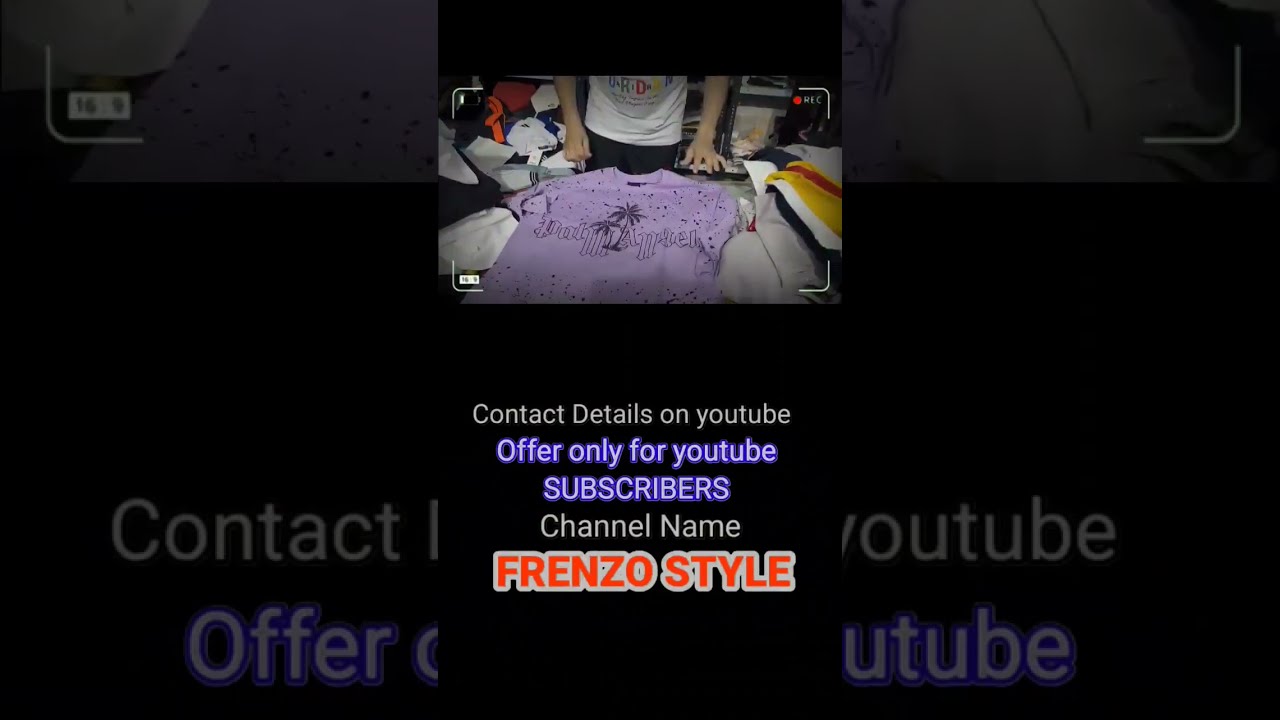The screenshot is an advertisement for a YouTube channel named "Frenzo Style." The top part of the image has a slightly blurry, dark border with white edges, suggesting it's a recording. The focal point is a partially visible male figure, visible from the chest to the waist, wearing a white shirt and black pants. In front of him lies a purple T-shirt adorned with a palm tree design and text that appears to read "Palm Angel." Surrounding the central image, the same scene is zoomed in and darkened, creating a layered effect. The table in the scene is cluttered with various other shirts. Below the image, in white text, it reads "Contact Details on YouTube," followed by "Offer Only for YouTube Subscribers" in prominent purple text, with "Subscribers" in all caps. Further down, the words "Channel Name" appear in white, and "Frenzo Style" is highlighted in red text with a white outline.